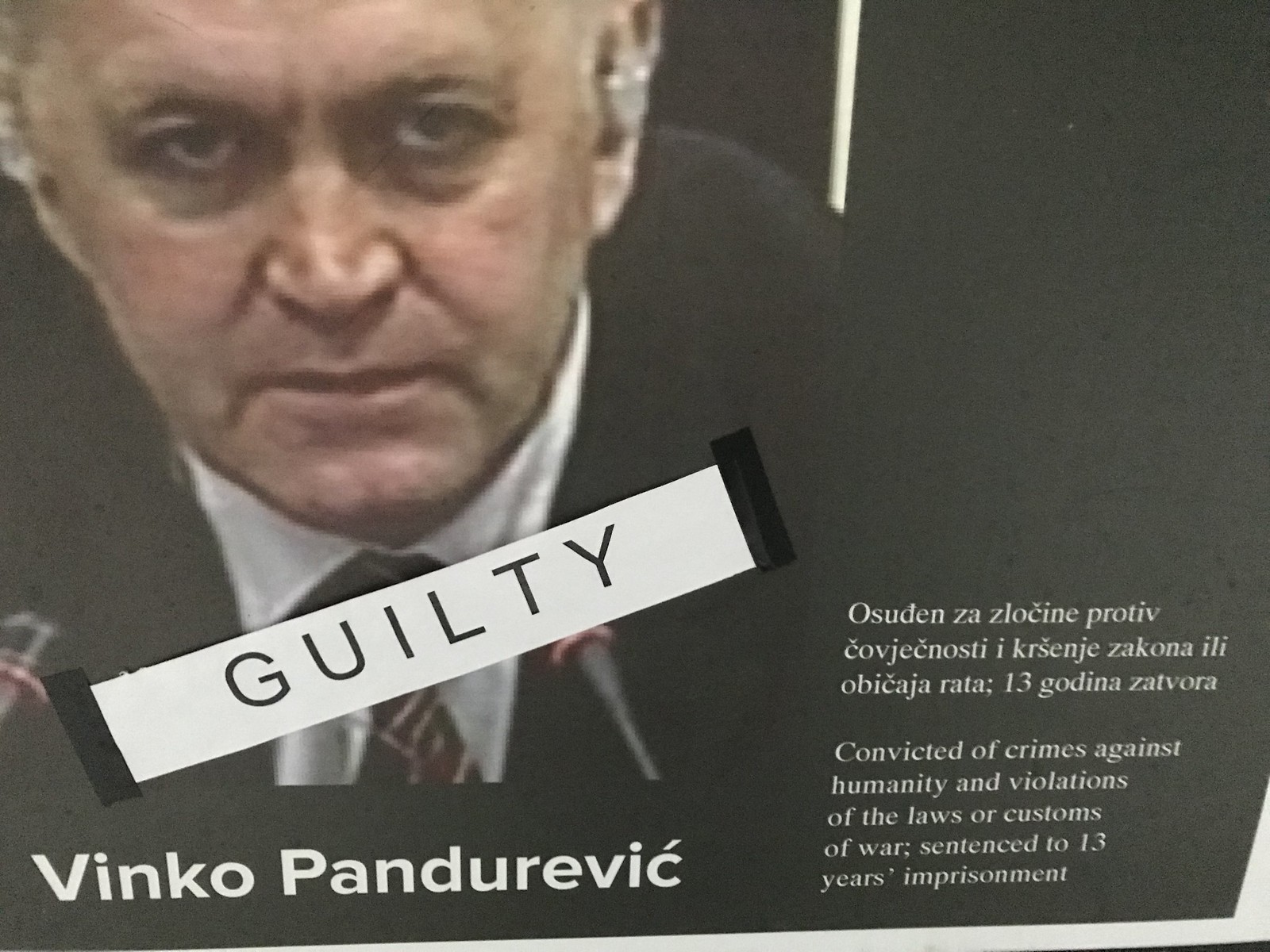This image, likely from a magazine article, shows a close-up photograph of an elderly man presenting as male, identified as Vinko Pandurovic. The man, with a stern expression, is dressed in a black suit, white shirt, and tie. Positioned in front of him are two small microphones, emphasizing a formal or judicial setting. Plastered across the bottom of the image, just below his chin, is a white strip with bold black letters reading "GUILTY." Beneath that, in white lettering, is the name "VINCO PANDEREVIC." The background is predominantly dark, adding to the somber tone of the image. On the bottom right, text in an Eastern European language is visible, partially legible as: "Ostuden za zoklin protiv kovrskni i krstnih zakona ili optika rata 13 godina rastova." In English, it translates to: "Convicted of crimes against humanity and violations of the laws and customs of war. Sentenced to 13 years imprisonment."